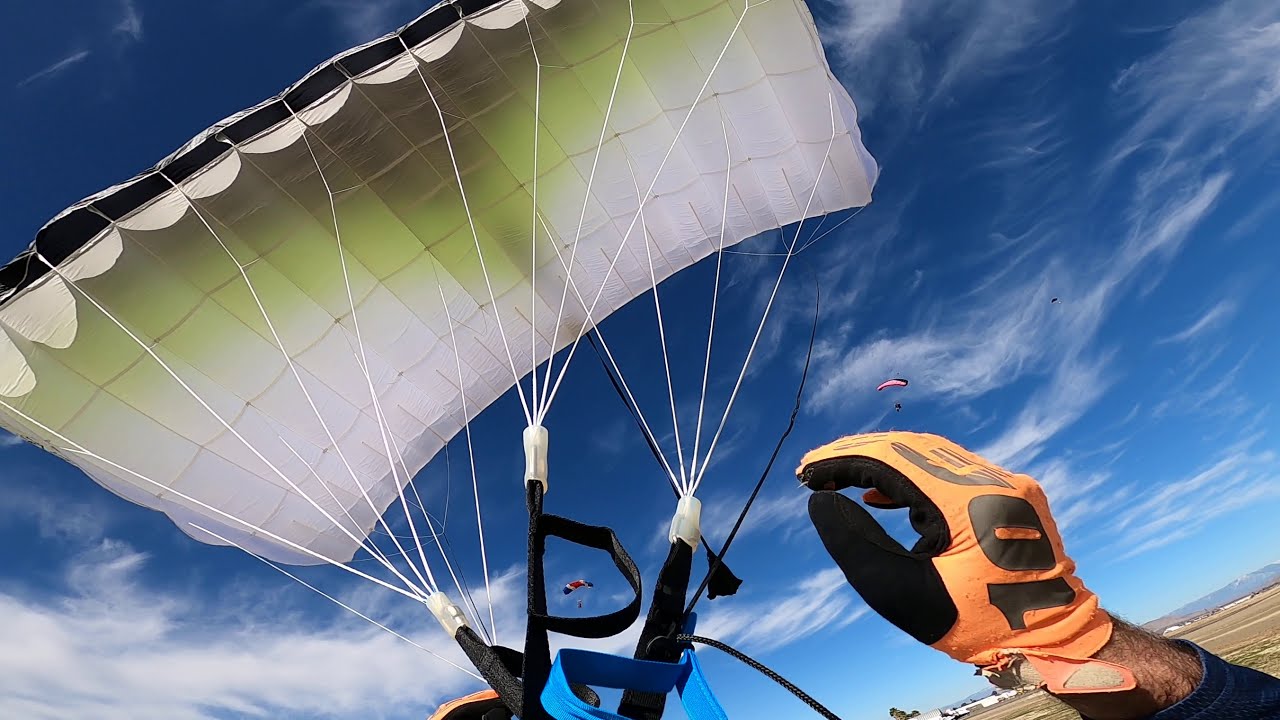This horizontally aligned rectangular image captures a thrilling moment in the sky, centered on a parachutist taking a selfie. The person, whose face is not visible, wears an orange and black glove on their right hand, marked with the number 10 and a logo. The camera is held in their left hand, while their right hand points up toward a white parachute with numerous strings attached to black handles. The bright blue sky is dotted with feathery white clouds and hosts other parachutists in the background. Three additional parachutists can be seen: one directly in front with a striped canopy, another to the right with a pinkish canopy, and two more tiny dots further up. A vast, distant landscape lies beneath them, possibly mountainous, suggesting an outdoor adventure venue. The scene, bright and seemingly mid-day, captures the exhilarating essence of parachuting against a serene, partially cloudy sky.